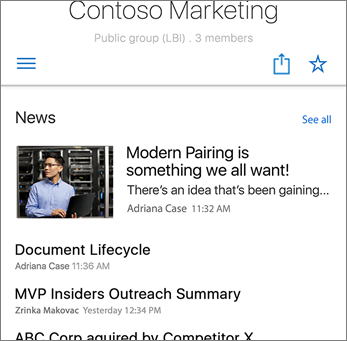**Websites Section**

In an extremely small image, the top prominently displays "Contesso Marketing." Below this header, the text indicates "Public Group LBI" with three members. The interface includes three iconic blue lines suggesting a navigational menu, an upload button, and a star button for favorites or important items. A dividing line separates the header from the content area below.

In the content section labeled "News," there is an image of a gentleman seated in what appears to be a server room, intently working on a laptop. He is wearing glasses and has dark hair and a blue shirt. His right hand is poised as if typing, and he gazes off to the left side of the image (his right).

Adjacent to this image is a headline that reads, "Modern Pairing is something we all want. There's an idea that has been gaining..." by Adriana Case, timestamped at 11:32 a.m. Following this headline are two more entries: "Document Lifecycle" by Adriana Case at 11:36 a.m., and "MVP Insiders Outreach Summary" by Shrinka Makovac, posted yesterday at 12:34 p.m.